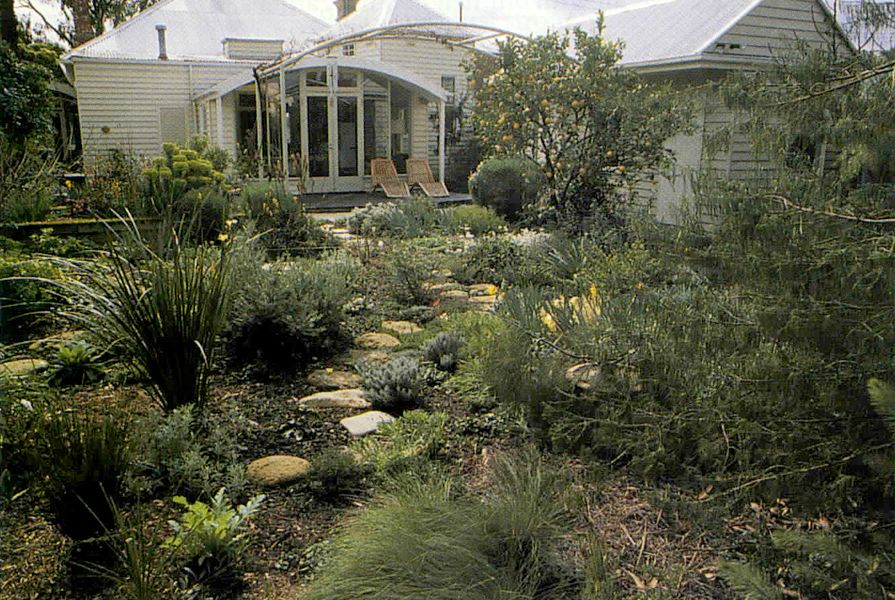This photograph showcases the front exterior of a house and its lush garden area. The bottom and foreground feature a vibrant garden filled with a variety of plants and bushes, all green and thriving. Among these, several small and taller trees can be seen, including a lemon tree full of lemons towards the middle back of the image. A narrow, uneven stone path winds its way through the garden, leading up to the front of the house.

The house itself is painted white and has a distinctive triangular roof. The exterior appears to have a metal or similar finish. At the front, there's a white overhang or archway providing a welcoming touch. On the patio, two tan lawn chairs are arranged, suggesting a cozy spot to relax. To the right of this house, another similar white house can be observed, continuing the serene suburban scene.